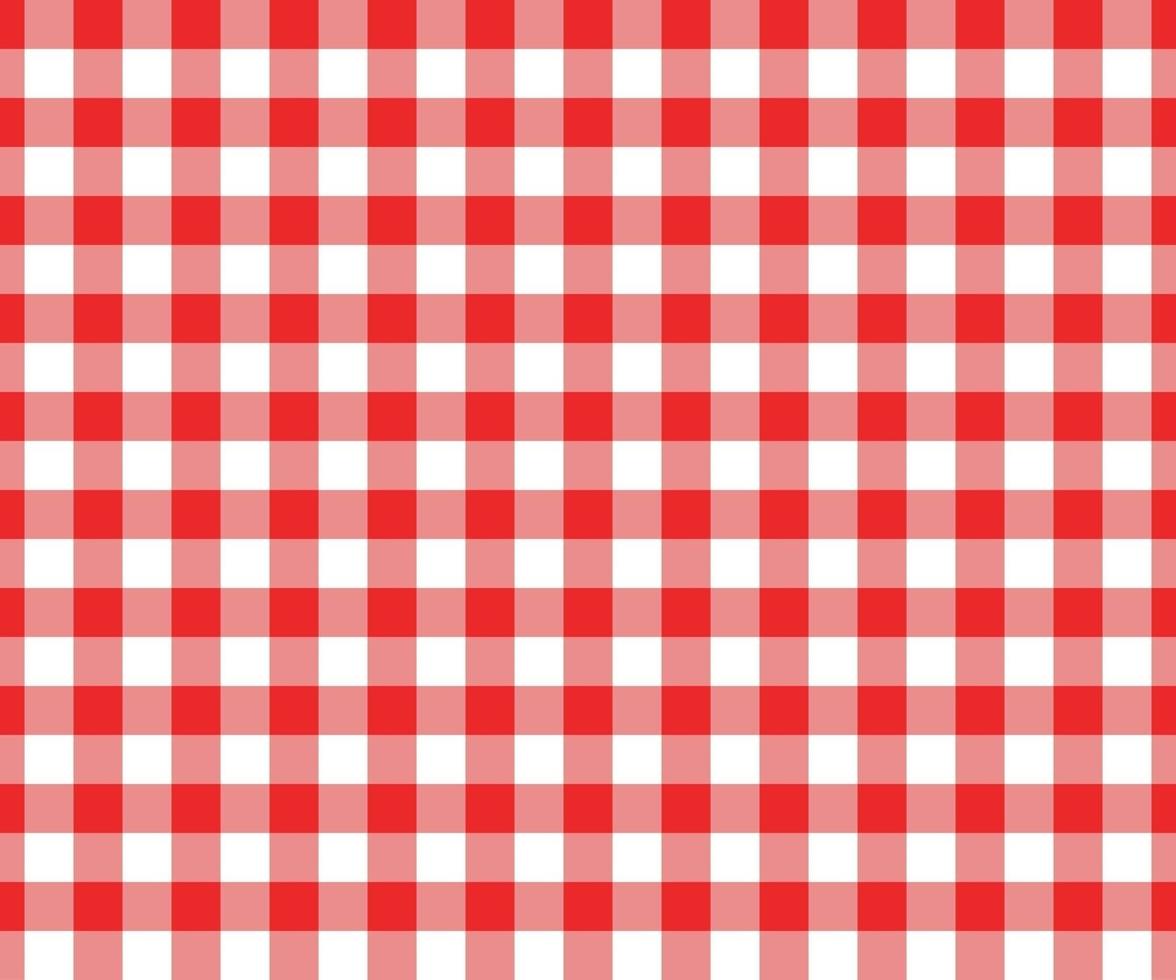The image is a detailed, digitally rendered checkerboard pattern consisting of three distinct colors: dark red, light pink, and white. The pattern alternates both horizontally and vertically. Horizontally, the rows follow a systematic sequence with dark red squares followed by light pink squares, followed by white squares. Vertically, the pattern aligns to create intersecting points where the colors mix: the intersections of dark red and light pink squares form additional red squares, creating a rich, layered aesthetic. Overall, the captivating design features about 400 squares, making up a consistent 20 by 20 grid that captures a visually appealing and repetitive arrangement without any textual overlay. The entire composition highlights a methodical blend of colors and geometric precision, resulting in a simple yet intricate visual experience.